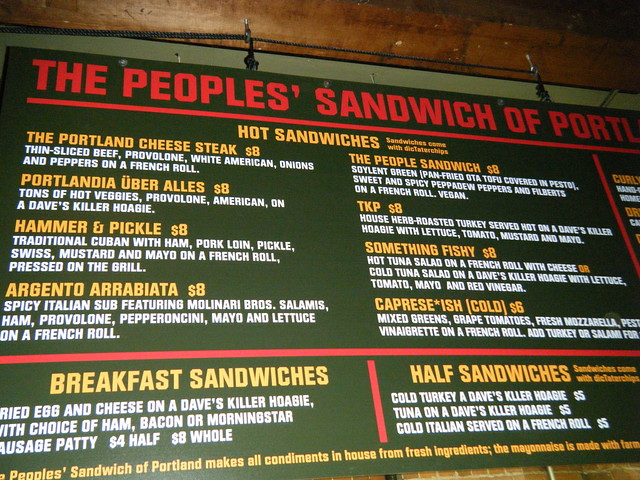The image features a wall adorned with brown wood trim and painted a greenish hue. At the top of the wall, several hooks are lined up, supporting a large blackboard-style menu. Prominently displayed, the menu announces "The People's Sandwich of Portland" in striking red letters, underlined by a bold red line. Beneath this heading, "Hot Sandwiches" is highlighted in yellow letters. The menu lists a variety of sandwiches, each priced at $8.00: 

- Portland Cheese Steak
- Portlandia Uber Alley's
- Hammer and Pickle
- Argento Arrabiata
- The People's Sandwich
- TKP
- Something Fishy

Additionally, it offers a "Capricious Cold" sandwich for $6.00.

Further down, "Breakfast Sandwiches" appears in yellow letters, followed by a detailed description in white. It features a "Fried Egg and Cheese on a Dave's Killer Hoagie," available with a choice of Ham, Bacon, or a MorningStar Sausage Patty. This breakfast offering is priced at $4.00 for a half and $8.00 for a whole sandwich.

On the other side of the menu, "Half Sandwiches" is labeled in yellow. The options include:

- Cold Turkey on Dave's Killer Hoagie
- Tuna on Dave's Killer Hoagie
- Cold Italian, served on a French Roll

The detailed, painted menu showcases an inviting array of artisan sandwiches, highlighting different combinations and price points, all set against the backdrop of a well-decorated wall.